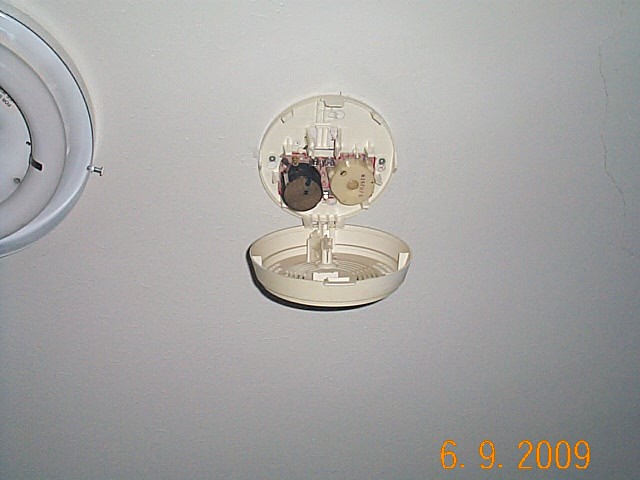This color photograph depicts an open smoke alarm mounted on a white plaster wall. To the left of the smoke alarm, there is a circular fluorescent ceiling light with a visible silver screw protruding from its left side. The smoke alarm appears to have its front cover removed, revealing its internal components and red wiring. In the bottom right corner of the image, an orange date, "6. 9. 2009," is clearly visible, with spaces between each of the numerals.